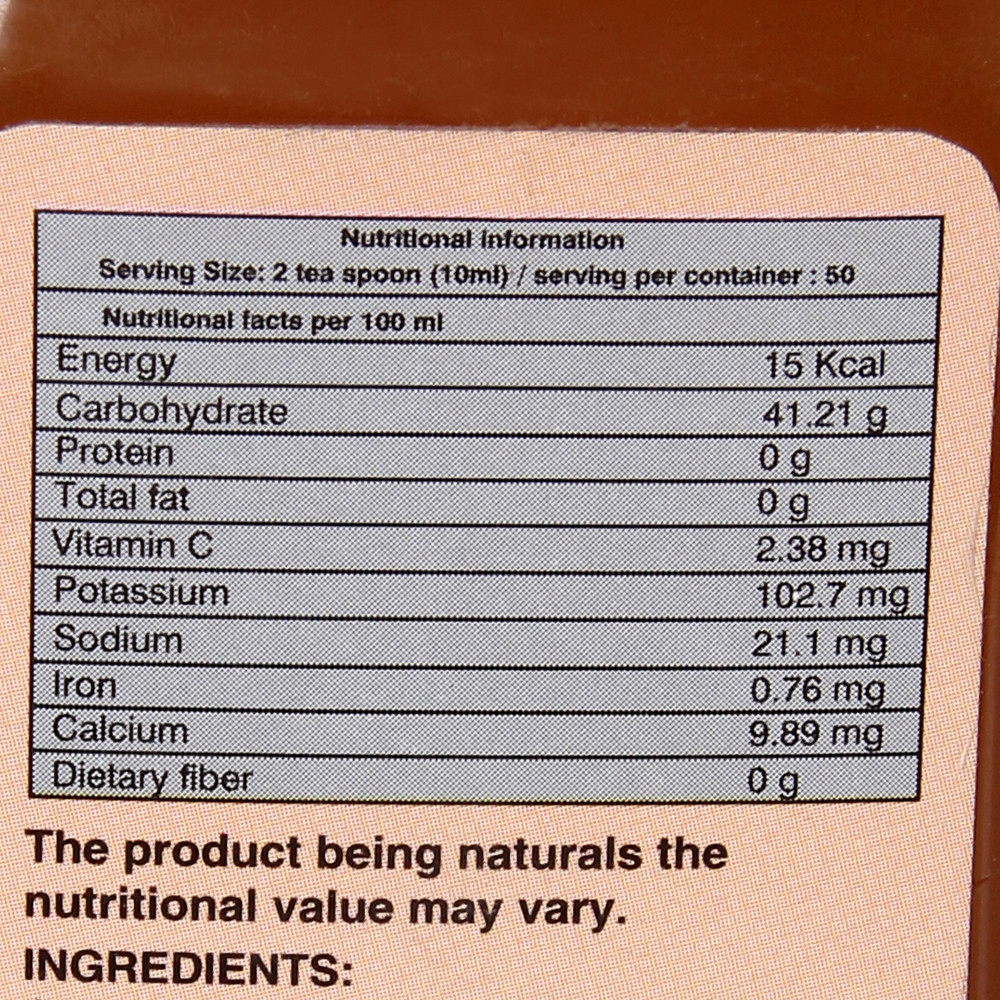This is an extremely close-up image of a food product's nutritional information label, dominating the frame. The label is situated on a food packaging box that exhibits a rusty brown color at the top. The label itself is a light pink, while the nutrition facts are displayed within a light blue box with black text. The label details the following:

- **Nutritional Information**
  - **Serving Size**: 2 teaspoons
  - **Energy**: 15 Kcal (uncommon notation)
  - **Carbohydrate**: 41.21 grams (precise measurement, usually rounded)
  - **Protein**: 0 grams
  - **Total Fat**: 0 grams
  - **Vitamin C**: 2.38 milligrams
  - **Potassium**: 102.7 milligrams
  - **Sodium**: 21.1 milligrams
  - **Iron**: 0.76 milligrams
  - **Calcium**: 9.89 milligrams
  - **Dietary Fiber**: 0 grams

Beneath these metrics, a disclaimer in black text reads: "Being naturals, within us, the nutritional value may vary." The label concludes with the heading "Ingredients:" visible at the bottom edge of the image.